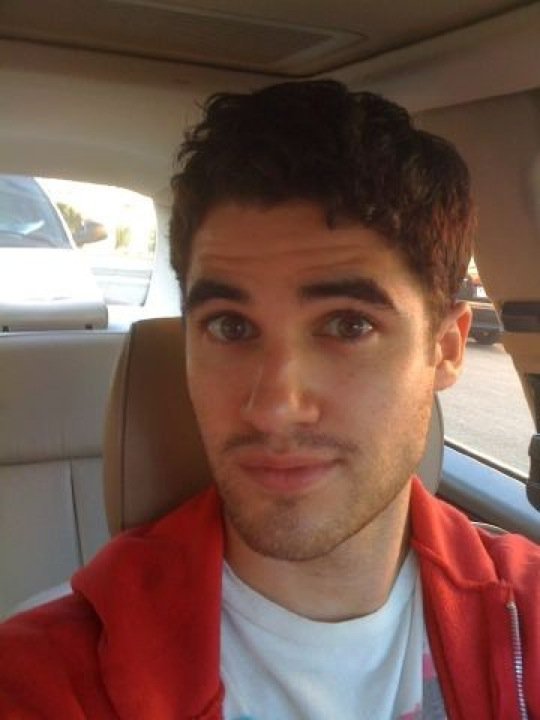A young man, possibly in his mid-20s and with an appearance that could pass for an actor, is pictured taking a selfie in his car, presumably while stopped in traffic or at a stoplight. He has short, messy black hair cut above his ears, complemented by bushy black eyebrows and a lightly scruffy beard. His large brown eyes gaze directly into the camera with a subtle smile on his face. He's dressed in an orange (or perhaps red) zip-up hoodie over a white t-shirt with some red and black prints visible. The car has a beige leather interior with seats and an off-white upper section, partially visible through a closed sunroof. The scene appears to be during daylight hours, and the car, a four-door model, indicates a modern, comfortable vehicle. There is a hint of another car visible behind his, suggesting a possible traffic jam or parking lot scenario.